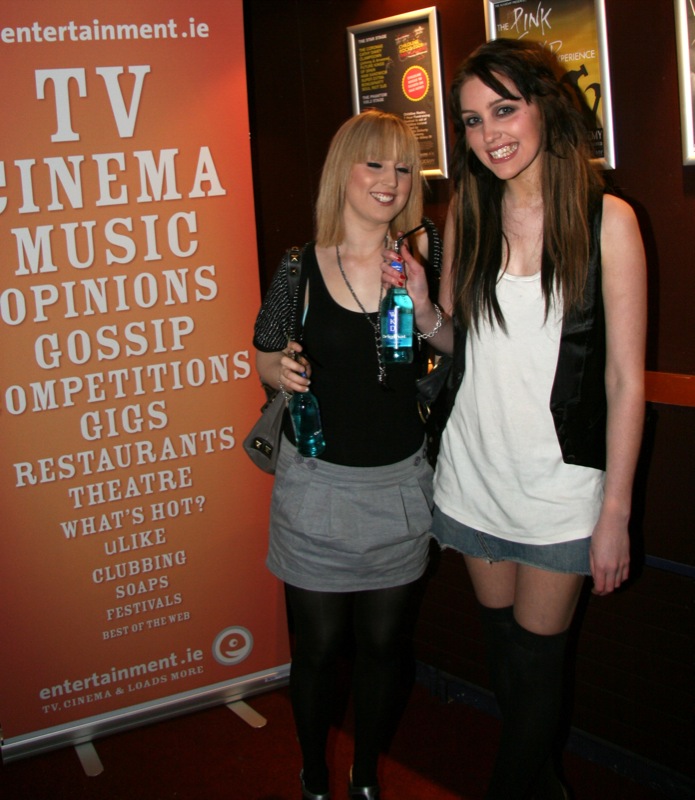This image features two young women standing next to a large, vertical, orange pop-up banner that is taller than they are. The banner prominently displays the text "Entertainment.ie" and lists various forms of entertainment such as TV, cinema, music, opinions, gossip, competitions, gigs, restaurants, theater, what's hot, clubbing, soaps, festivals, best of the web, and loads more. At the base of the banner is a circular logo with a stylized "E" that has an eye inside it. 

The woman on the left, who is shorter, has blonde bangs and shorter hair. She is dressed in a white tank top, a gray skirt, black leggings, and black shoes. She has a toothy smile and is holding a blue beer bottle labeled "WKD." The taller woman on the right has long brown hair reaching down to her chest. She is smiling broadly, showing all her teeth, and appears to have either a retainer or Invisalign, with pink lipstick accentuating her smile. She is wearing a sheer black vest over a white tank top, short jean shorts, and thigh-high black boots. She also holds a blue WKD drink bottle in her right hand.

Both women are smiling, though the blonde woman is caught mid-blink, and behind them is a maroon wall adorned with indistinguishable movie poster-like signs.